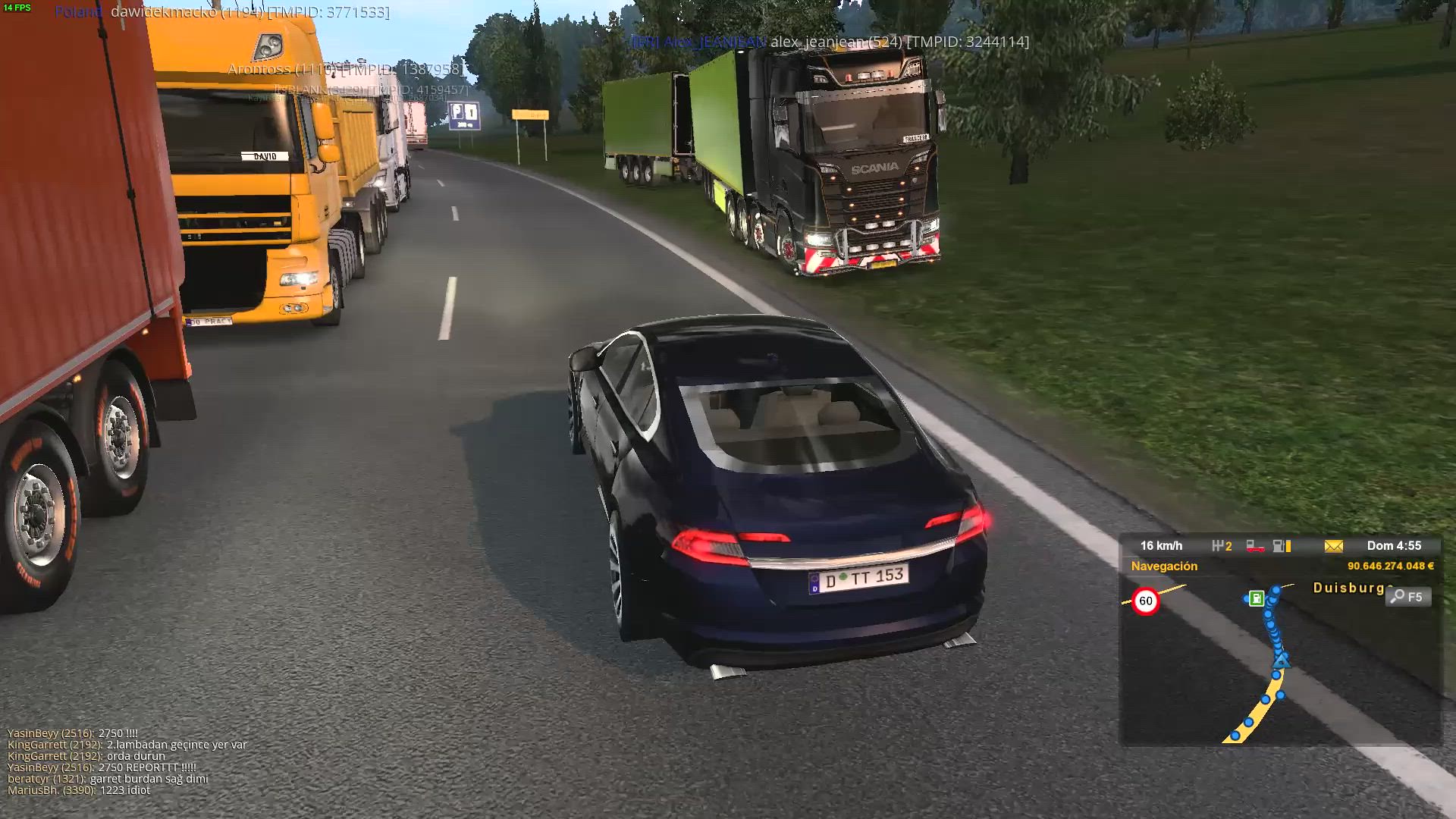In this computer-animated in-game screenshot from a driving simulator, a purple sports car is seen driving straight in the right car lane. To its right, parked on a lawn, is a black and green semi truck. On the left in the opposite lane, there are three semi trucks in sequence: a red one, followed by an orange one, and lastly a white one. The scene is populated with trees in the background and roadside signs, including a yellow one and a blue-and-white one. The image also features game interface elements; in the bottom right corner, there is a mini-map displaying the navigation route, speed, and fuel levels, while the top left corner shows an FPS counter indicating the game is running at 14 frames per second.